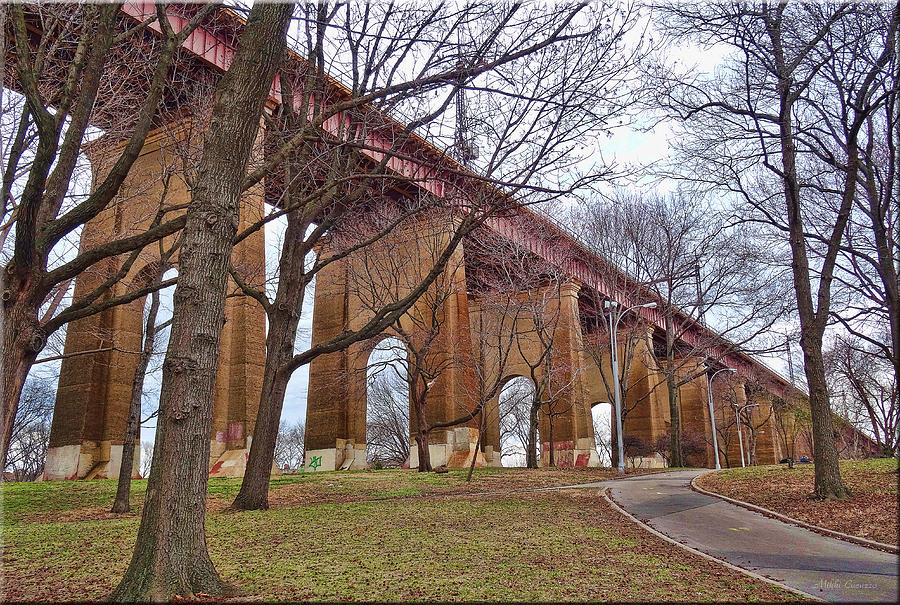The photograph captures a detailed view of an elevated roadway bridge, characterized by its architecturally intriguing arched supports made of a dark, rusty brown stone or brick material. Each support structure features a distinctive dome-shaped cutout in the center, possibly to allow passage through. The bridge spans diagonally from the top left corner to the bottom right, standing tall over a park area. The bridge's superstructure displays a reddish metallic color, contrasting with the brownish concrete base. Below the bridge, the vibrant yet patchy green grass of the park is interspersed with brown areas, likely due to the winter season, as evidenced by the leafless tall trees with long branches and the overcast sky. A winding gray pathway, adorned with street lamps on the left, traverses the park, leading towards a small street beneath the bridge that allows driving through. Scattered brown and orange leaves cover the ground, accentuating the seasonal atmosphere.